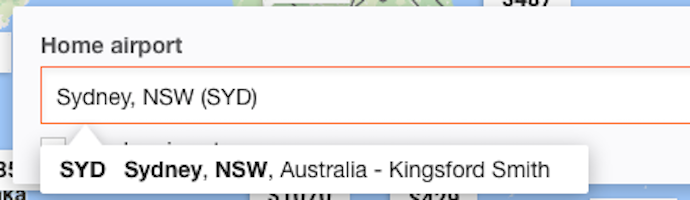The image features a bluish background that appears to resemble a map. Scattered across the background, there are touches of green and white, hinting at terrain and possibly clouds or other features. Superimposed on the map are several white boxes containing text or numbers, though these elements are largely obscured by a prominent white rectangle positioned atop them.

In the top left corner of this white rectangle, the phrase "Home Airport" is displayed. Adjacent to it, on the right, is an open-ended red rectangle—this shape is outlined in red on the top, left, and bottom edges while remaining open on the right side. Inside this red frame, the text reads "Sydney, NSW (SYD)."

An additional label stands out in the form of a white tab, shaped like a rectangle topped with a small triangle. This tab contains the text "SYD Sydney, NSW, Australia-Kingsford Smith."

The map appears incomplete or cut off at the bottom, left, and top edges, while the right side of the image is entirely blank, save for the text and shapes already described.